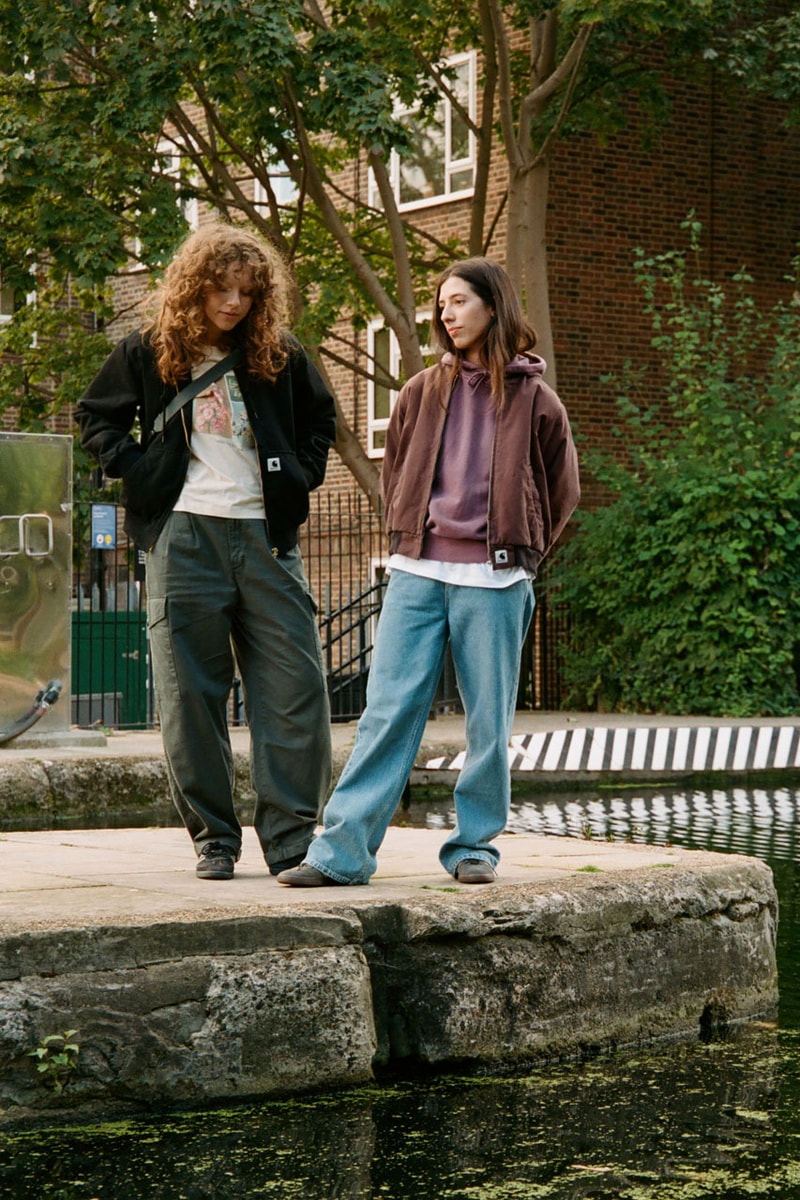In this photograph, two young women stand on a small stone ledge that juts out over a pond with greenish, algae-speckled water. The woman on the left, who has long curly reddish-brown hair, is wearing a black jacket over a white t-shirt with some design in the middle, paired with baggy dark green cargo pants and black shoes. She has a bag that runs across her chest and is looking down. The woman on the right has long brown hair and is dressed in a brown jacket over a maroon sweatshirt and a purple sweater, with a long white t-shirt showing underneath. She is also sporting light blue jeans and black shoes, and stands with her hands behind her back, looking to the left. 

The backdrop features a partly obscured brick building with white-bordered windows, framed by a tree with dark green foliage and a bush with similarly dark green leaves to the right. The scene evokes a tranquil setting with these young women poised thoughtfully on the edge of the pond, surrounded by the serene natural elements and the rustic architecture.